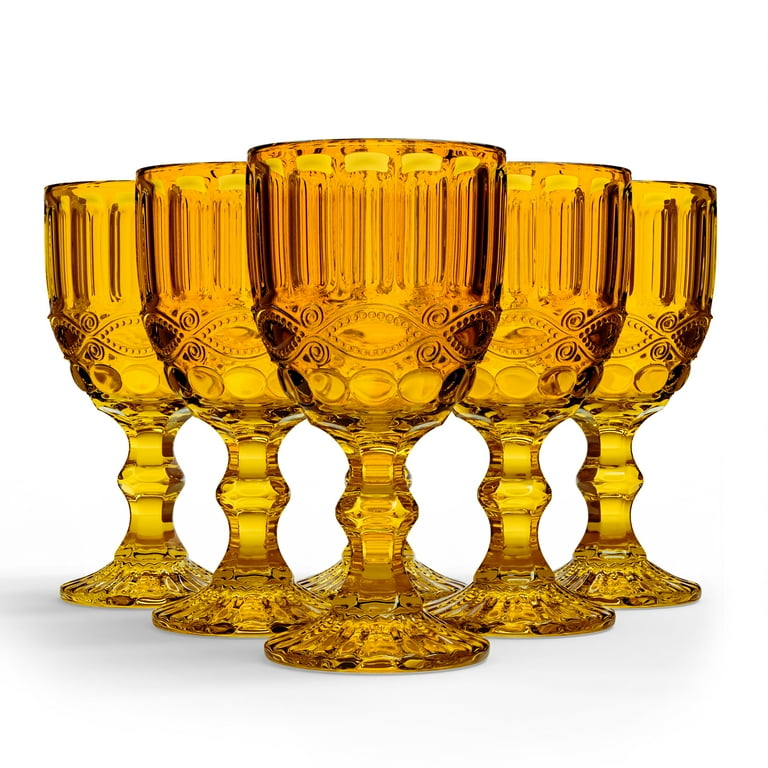This striking photo showcases six intricately designed amber or gold glass goblets, arranged meticulously in a pattern reminiscent of bowling pins. At the forefront stands a single goblet, followed by two more positioned slightly further apart behind it, and another set of two spaced even wider apart, forming a neat triangular formation. The goblets rest on a pristine white surface against a uniformly white backdrop, emphasizing their ornate detailing and warm hue. The elegant glassware, likely being advertised in this image, features exquisite ridges on the rims, curly and ornate embellishments encircling the middle, and circular motifs adorning the base. The stems are gracefully wide and curved, with additional curlicue designs enhancing the bottoms, showcasing the meticulous craftsmanship that went into their creation.